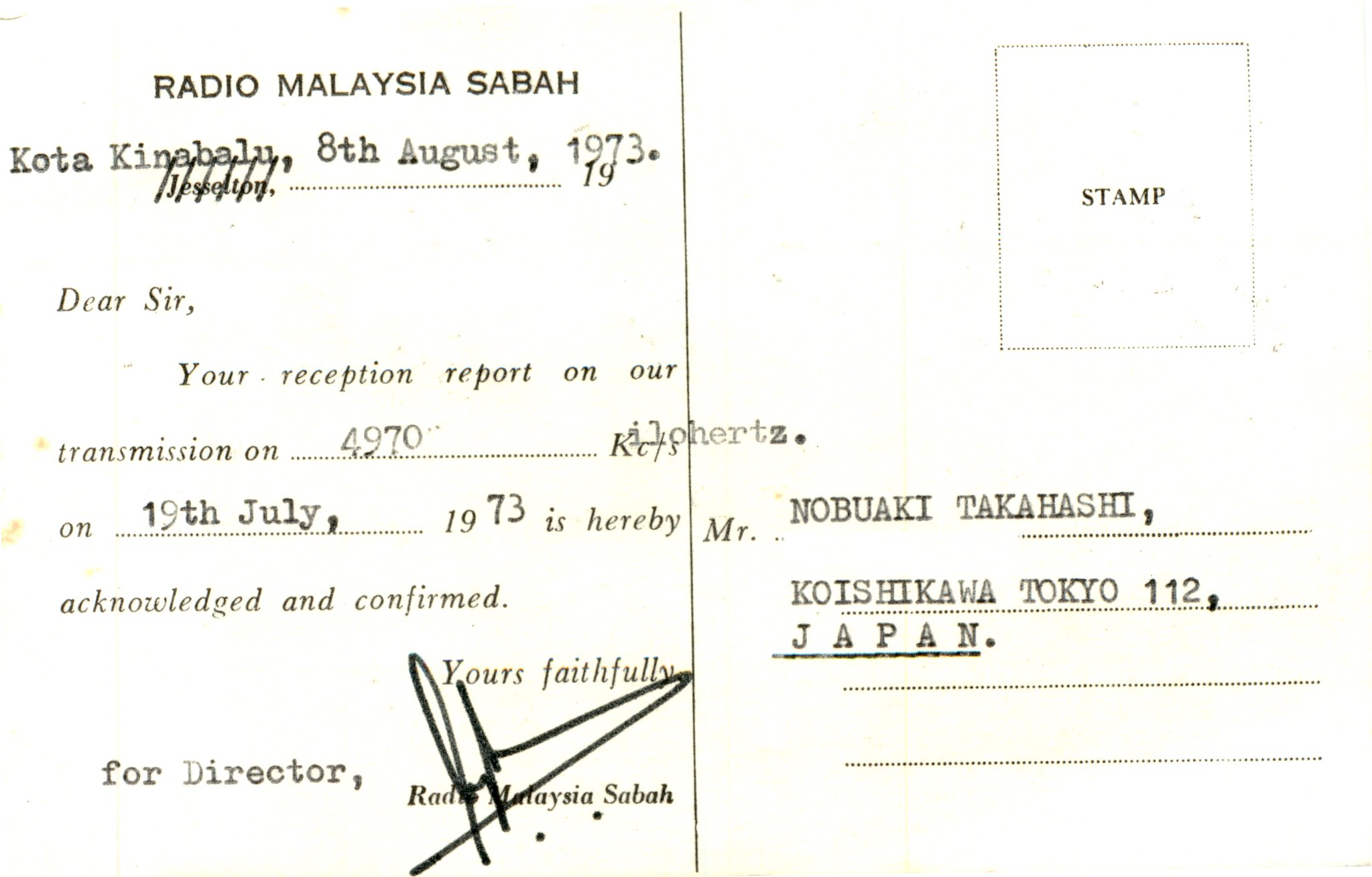The image is of a rectangular postcard with a yellowish off-white background. On the right side, there is a vertically aligned dotted rectangle labeled "STAMP" in all capital letters, black text. Beneath this, typed over four dotted lines, the recipient's details read: "Nobuaki Takahashi, Koishikawa, Tokyo, 112, JAPAN." A vertical line runs down the middle of the postcard, separating the recipient's information from the message on the left. At the top left corner, in all caps, it says "Radio Malaysia Sabah." Below that, it is stamped "Kota Kinabalu, 8th August, 1973." The typewritten message reads: "Dear Sir, your reception report on our transmission on 4970 kilohertz on 19th July, 1973 is hereby acknowledged and confirmed. Yours faithfully, for Director, Radio Malaysia Sabah," followed by a scribbled signature.